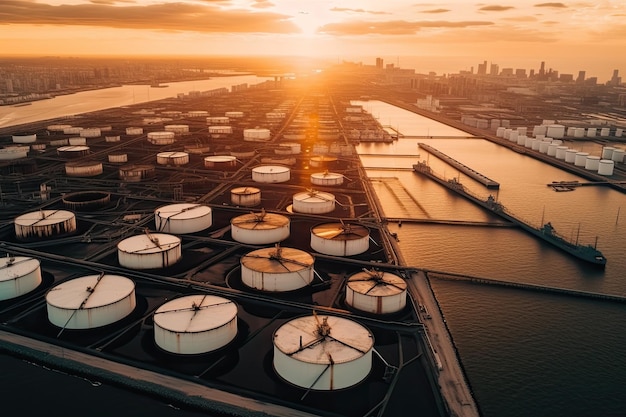The photograph captures an aerial view of a bustling dockside and cityscape at sunset. Dominating the center of the image are numerous large, white cylindrical silos positioned on a long dock that stretches towards the horizon. These silos are flanked by rectangular strips of water on either side. To the right of this central dock, more silos are visible across the water, while the center area features empty receptacles where additional silos could be installed. Surrounding these structures are several extending piers and a ship positioned centrally. In the distance, a sprawling city skyline emerges against a dramatic backdrop of dark clouds and an orange-tinged sky. The setting sun hangs low, casting a brilliant reflection off the water and suffusing the entire scene with a warm, golden glow.